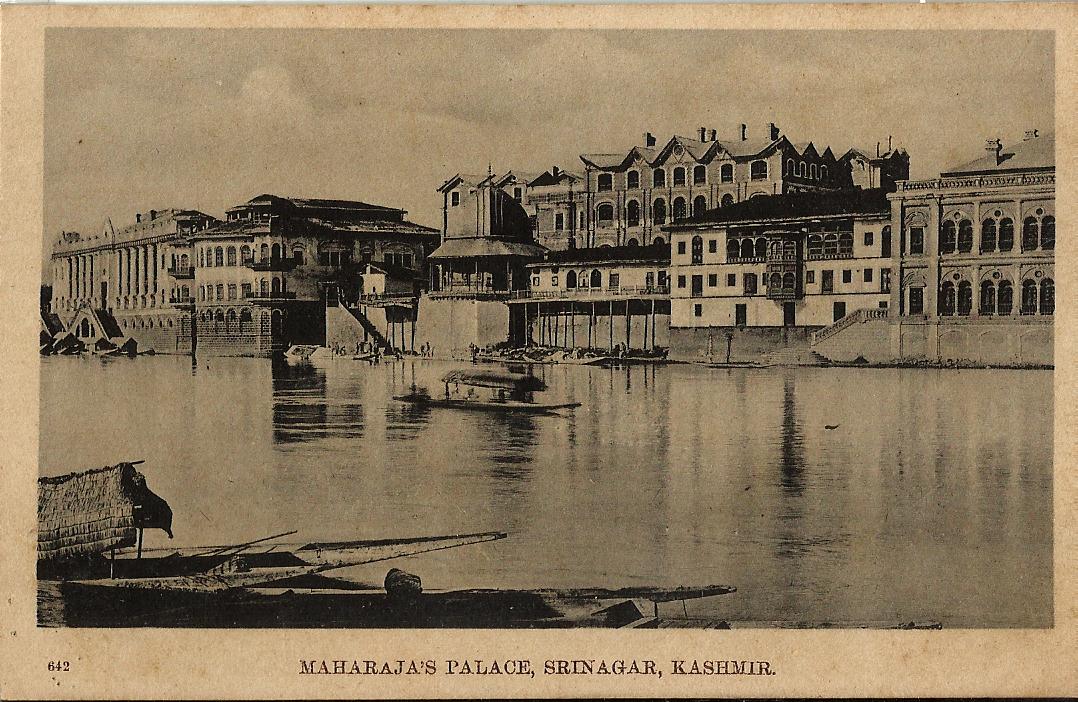This vintage black and white photograph, labeled "Maharaja's Palace, Srinagar, Kashmir," captures a picturesque scene in India. The image, with a light brown and beige tint suggesting its age, features a series of buildings lined up along the shoreline, mirrored in the serene body of water that separates them from the viewer. Prominent architectural elements like peaked roofs, chimneys, and numerous windows detail these structures, hinting at their historical significance and possibly even an industrial past. Dominating the scene is a boat in the foreground, its reflection visible in the water, adding a layer of tranquility. The sky is cloudy, enhancing the vintage, almost sepia-toned ambiance of the photograph. The photograph's border is a faint, aged brown, and the bottom left corner is marked with the number 642, adding to its antique charm. Although undated, the overall aesthetic strongly indicates its considerable age, offering a nostalgic glimpse into a bygone era.